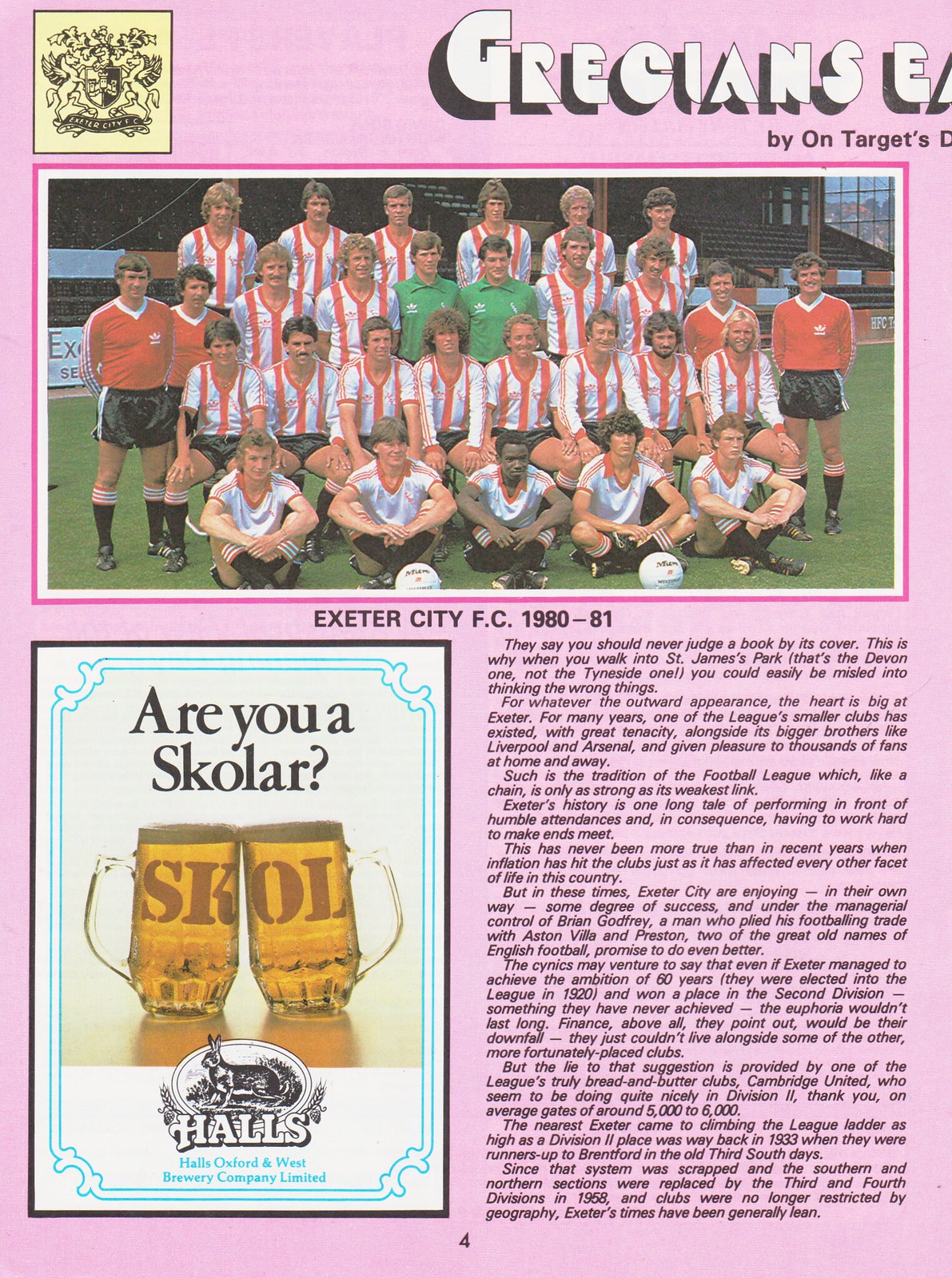This vertically aligned rectangular image, likely clipped from a newspaper or magazine, features a light purple background. Dominating the upper section of the image is the partially cut-off header "Grecians", positioned in bold white block letters. Below this, the text "buy on targets" appears, though it is also partially cut off. On the top left corner, there is a square logo with a black emblem set against a yellow background.

The central portion of the image showcases a historic photograph of the Exeter City FC soccer team from the 1980-1981 season. This team is organized into four rows: the front row consists of players sitting cross-legged, the second row is kneeling, the third row is standing, and the back row is also standing. The players predominantly wear red and white striped jerseys. Notably, two individuals in green shirts are positioned in the middle, with coaches in red tops on each end.

Below the team photograph, on the lower right-hand side, there is a dense column of fine print detailing the soccer team's achievements and information. On the lower left-hand side, there is a vertical rectangle bordered with blue lines. This section features an advertisement that asks, "Are you a skolar?" spelled out as S-K-O-L-A-R, accompanied by an illustration of two beer mugs clinking. This advert is associated with 'Halls Oxford and West Brewery Company Limited'. At the very bottom center, the page number '4' is displayed, indicating the source page of this clipping.